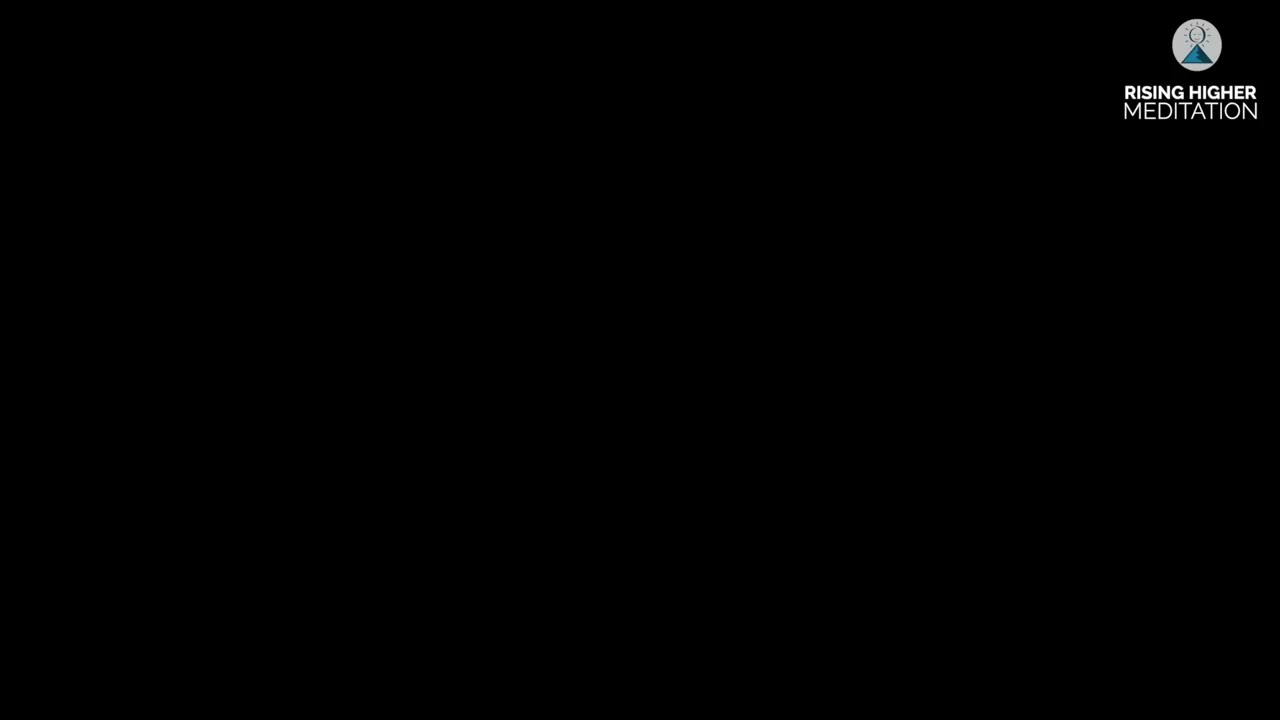The image features an extremely minimalistic design with a solid black background filling the majority of the rectangular frame. In the upper right corner, there's a small logo composed of a white circle containing a blue pyramid. Above the pyramid is a simplistic illustration of a sun with radiating lines, which could be interpreted as a smiling face. Directly beneath this graphic element, the text "RISING HIGHER MEDITATION" is written in white, all-caps typography, spanning two lines. The logo and text are the only elements within the image, giving it an appearance akin to an ending slide of a presentation or possibly an advertisement for a meditation service. The overall color palette is predominantly black, accented by shades of white, gray, and a blue-green hue within the logo.